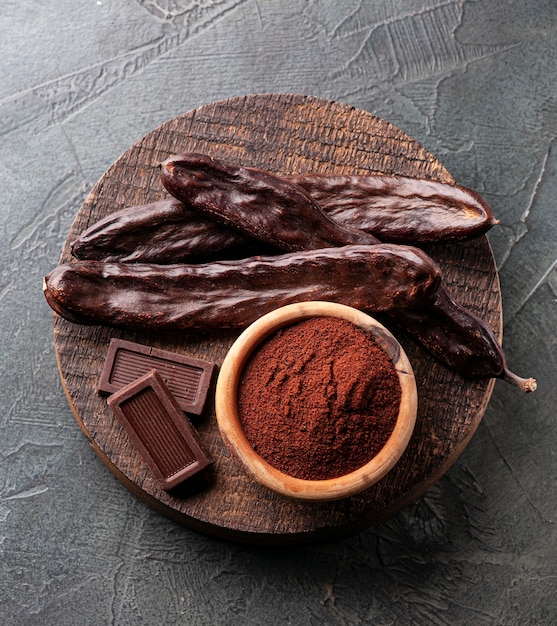The top-down photograph captures a culinary arrangement on a deep brown wooden circular platter, set against a textured dark gray table surface with visible ripples and lines. The centerpiece consists of three elongated, dark brown cocoa pods arranged in varying orientations—two horizontal and one diagonal. Nestled below the cocoa pods is a light brown ceramic bowl filled with a rich, dark red powder, presumably ground cocoa. To the left of the bowl, two small dark chocolate bars, each adorned with horizontal lines, complete the composition. The overall scene appears to illustrate the process and elements of cocoa and chocolate preparation.